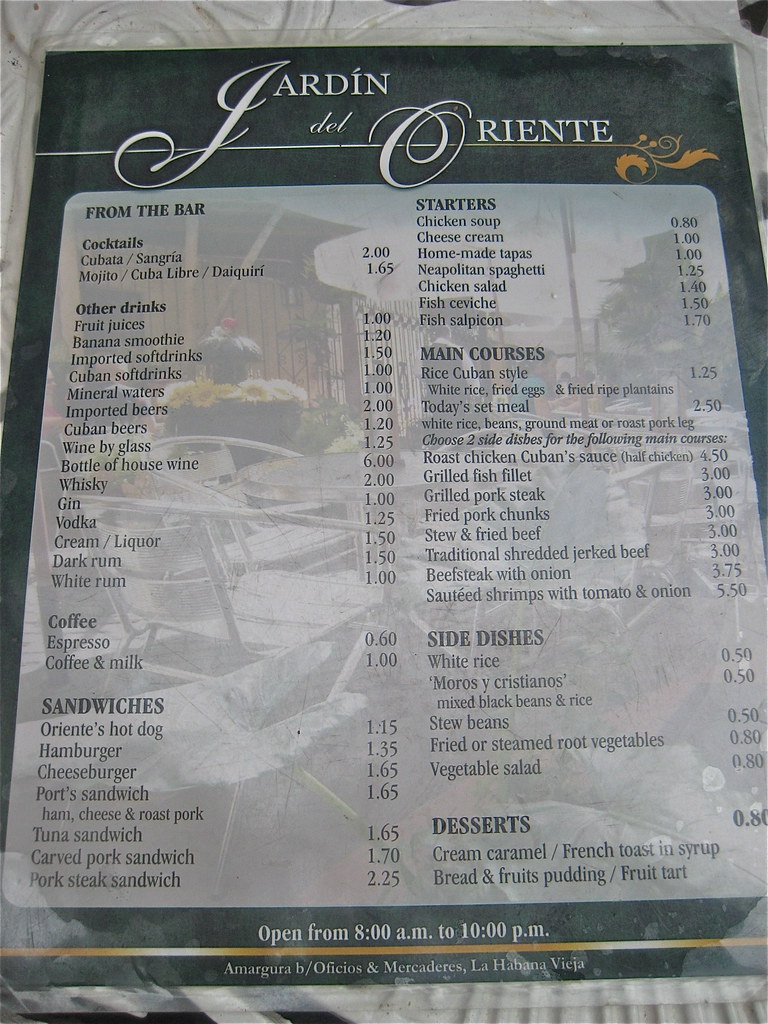This photograph captures the elegant menu of a sophisticated restaurant, "Jardin del Oriente," set against a pristine white tablecloth, with glimpses of an outdoor scene featuring flowers in the top left corner and a brown building in the background. The menu features stylish white lettering at the top, with the restaurant name "Jardin del Oriente" in a sophisticated font. To the right of the title, there's an ornate orange leafy design.

The main section of the menu is vertically oriented and lists various items in black lettering, starting with offerings from the bar, followed by starters such as chicken soup and chicken salad, each with its price indicated. The categories span drinks, sandwiches, side dishes, and end with desserts at the bottom. Below the menu items, there's an inscription in white indicating that the restaurant is open from 8 a.m. to 10 p.m., followed by a gold line. Further down, additional text appears in another language, potentially mentioning "bahia."

The entire menu is set against a subtly visible background image that appears to depict a pool or backyard area, adding to the luxurious and relaxed ambiance of the dining experience.